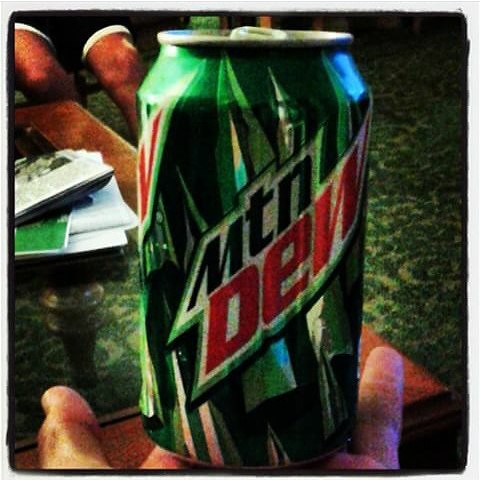In this vividly detailed image, a hand emerges from the bottom of the frame, clasping a green aluminum can of Mountain Dew prominently displaying the "MTN Dew" logo. The can stands out against the vibrant green carpet adorned with intricate designs. The fingers—index, middle, and ring—wrap around the can with the tab and silver ring clearly visible at the top. Below the hand rests a glass-top table framed with wood, scattered with magazines and papers. Across the room, legs clad in black shorts with a white hem are visible, adding a casual, lived-in feel to the scene.